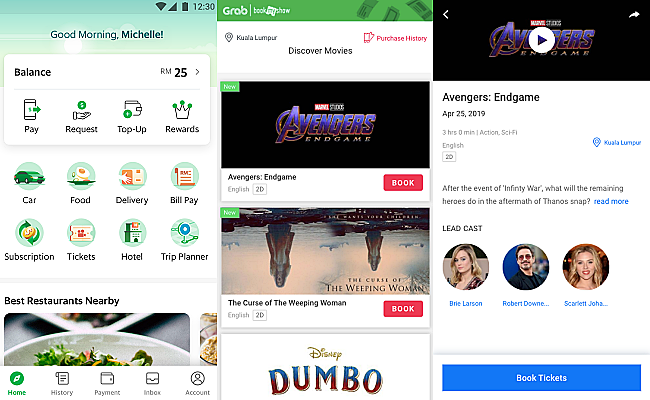A horizontally aligned composite screenshot of three phone screens:

1. **Left Screen**: 
   - Header: "Good morning, Michelle" on a green background.
   - Balance: Displays a balance of 25 RM.
   - Icons beneath the balance: "Pay," "Request," "Top up," and "Rewards."
   - Additional service icons: "Car," "Food," "Delivery," "Bill Pay," "Subscription," "Tickets," "Hotel," and "Trip Planner."
   - Section titled "Best Restaurants Nearby" featuring food photographs.
   - Navigation icons at the bottom: "Home" (highlighted in green), "History," "Payment," "Inbox," and "Account."

2. **Center Screen**: 
   - Website displayed: "Grab Book My Show."
   - Featured movie banners:
     - "Avengers Endgame" with a new green button.
     - "The Curse of the Weeping Woman" with a new label and an orange "Book" button.
     - Partial view of "Disney Dumbo."
   - Header: "Discover Movies" with a "Purchase History" section.

3. **Right Screen**: 
   - Featured banner again for "Avengers Endgame" with a play button to watch a video trailer.
   - Detailed movie information:
     - Title: "Avengers Endgame."
     - Show date and running time.
     - Location: "Kuala Lumpur" listed in blue.
   - Synopsis: "After the event of Infinity War, what will the remaining heroes do in the aftermath of Thanos' snap?"
   - Lead cast icons and names: Brie Larson, Robert Downey Jr., Scarlett Johansson.
   - Blue rectangle at the bottom with "Book Tickets" in white text.

Each screen provides a unique interface and set of functionalities, ranging from financial management and service bookings on the left, to movie ticket purchases in the center, and detailed movie information on the right.